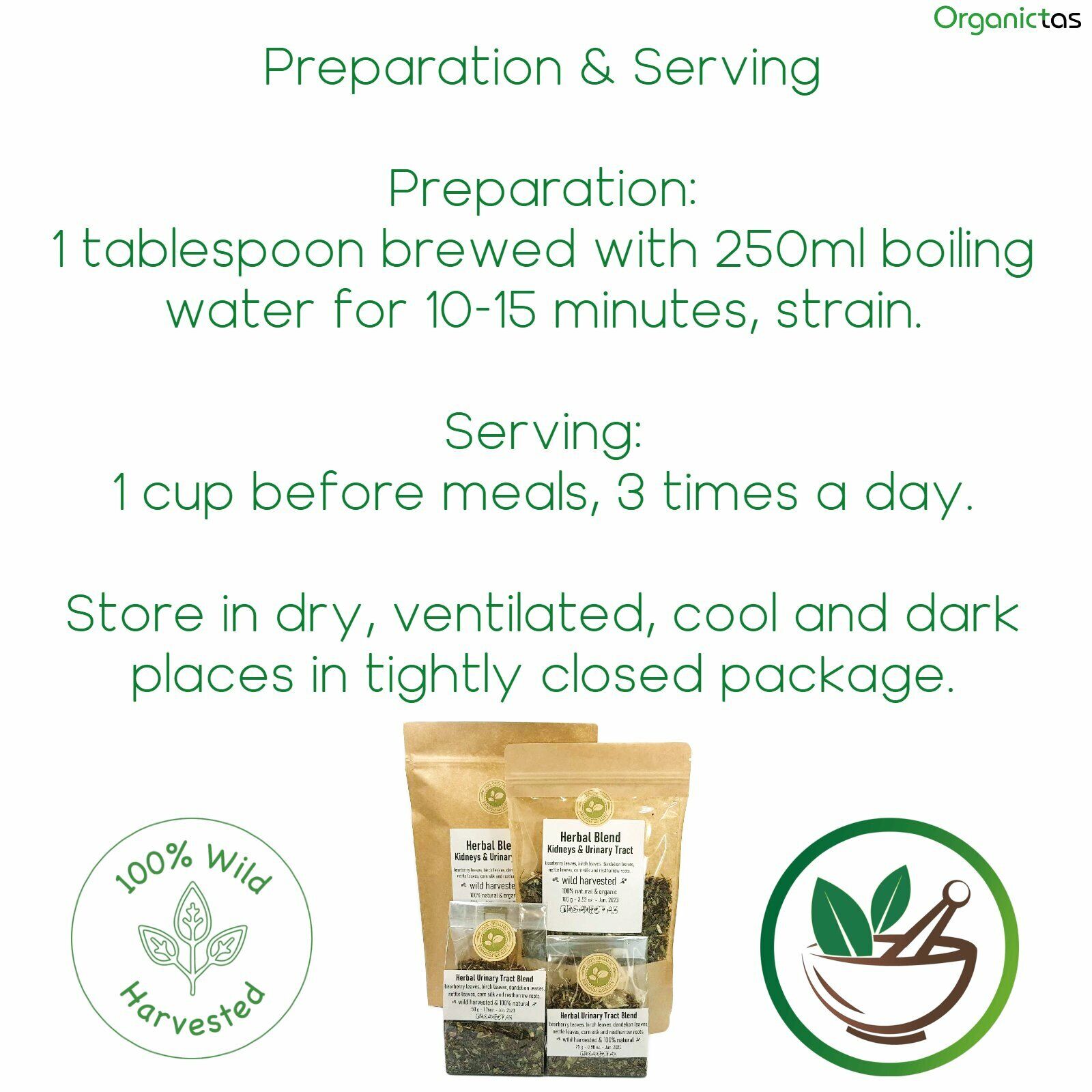This image features instructional text in green detailing how to prepare and serve an herb packet. The directions read: "Preparation and Serving: Use one tablespoon brewed with 250 milliliters of boiling water for 10 to 15 minutes, then strain. For serving, consume one cup before meals, three times a day. Store in a dry, ventilated, cool, and dark place in a tightly closed package." At the bottom of the image, there are various visual elements including the product itself, displayed in craft brown paper bags labeled "Herbal Blend Kidneys and Urinary Tract," along with a small plastic packaging containing herbs. On the left, a green circular logo states "100% Wild Harvested" and features three leaves. On the right, another green circular logo depicts a mortar and pestle with leaves, indicating the product is pharmaceutical plant-based. The overall background is white, and the top right corner features a logo that reads "Organic Toss."